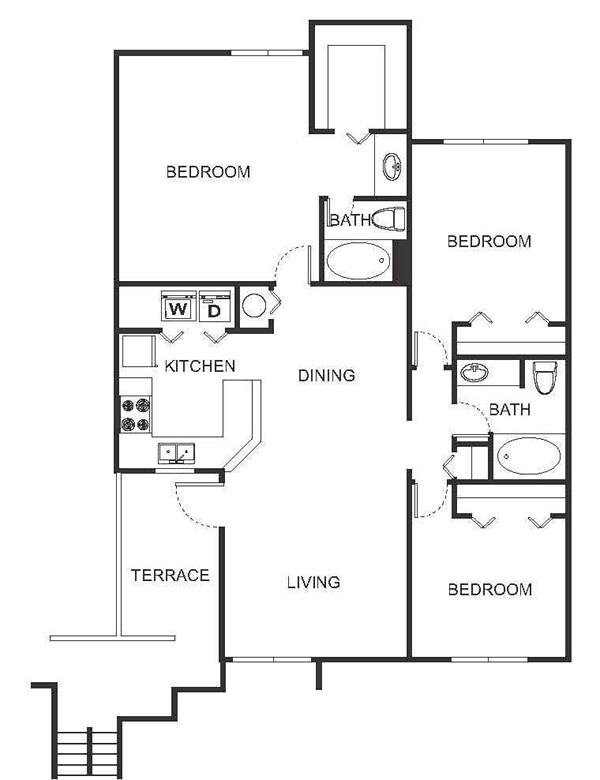This detailed floor plan of an apartment is presented in black ink on a white background. The diagram features a top-down view and employs various line styles, including solid, dotted, and thin black lines, to delineate different areas and elements.

In the bottom left-hand corner, the main entrance leads into a small room labeled "Terrace." Adjacent to the Terrace, a doorway on the right wall opens into the living room, which seamlessly connects to the dining room situated just beyond it.

To the left of the dining room is the kitchen, where the sink is positioned against the wall shared with the Terrace. The washer and dryer are located on the opposite wall in the kitchen, with the stove situated to the left of the sink.

Moving from the dining room towards the back of the apartment, there is a bedroom on the left. Adjacent to this bedroom, on the right, is an opening leading to a bathroom equipped with a sink, toilet, and bathtub.

To the right of the living room, another doorway provides access to a second bedroom if you turn right. Continuing straight through this doorway leads to another bathroom. If you turn left through this same doorway, you will find a third bedroom. This second bathroom offers access from both the second and third bedrooms, providing convenience and functionality.